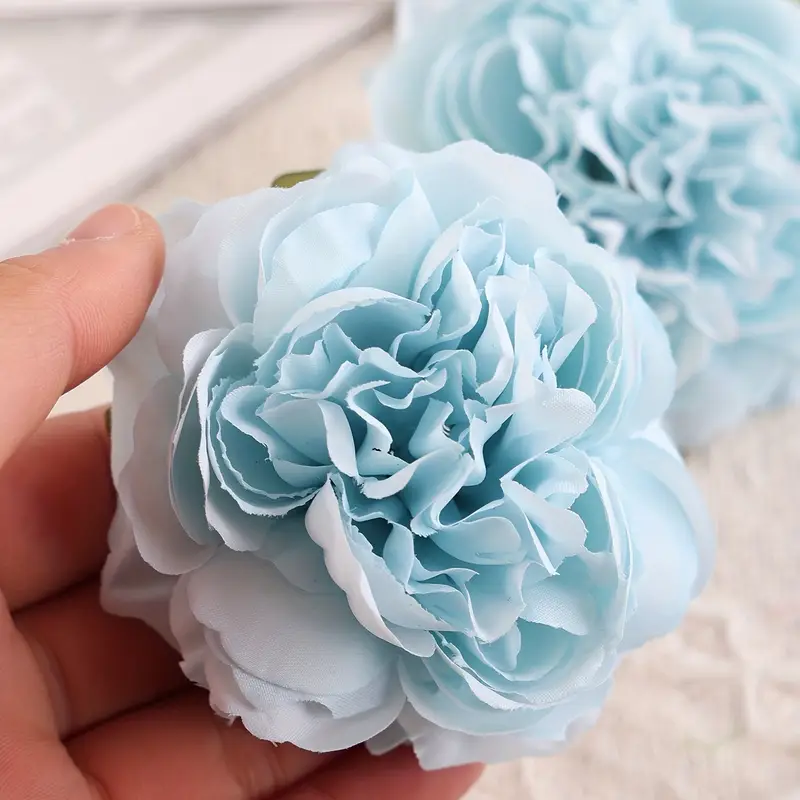In the photograph, a left hand, appearing young and pale, is prominently featured in the bottom left corner, gently holding a delicate, light blue flower. The flower, which appears to be synthetic and possibly made from cloth or thin paper, exhibits layers of petals that transition from blue at the center to white at the edges, resembling a carnation. The thumb is positioned on one of the petals, with the other fingers supporting it from underneath. Another similar blue flower lies beneath this hand, resting on a surface that could possibly be a tombstone, given the visible engraved text on a gray background. The hand seems to be placing the flower down next to its counterpart, suggesting a somber, maybe memorial setting. The overall background comprises beige tones, and the white surface beneath the lower flower creates a subtle contrast with the scene.